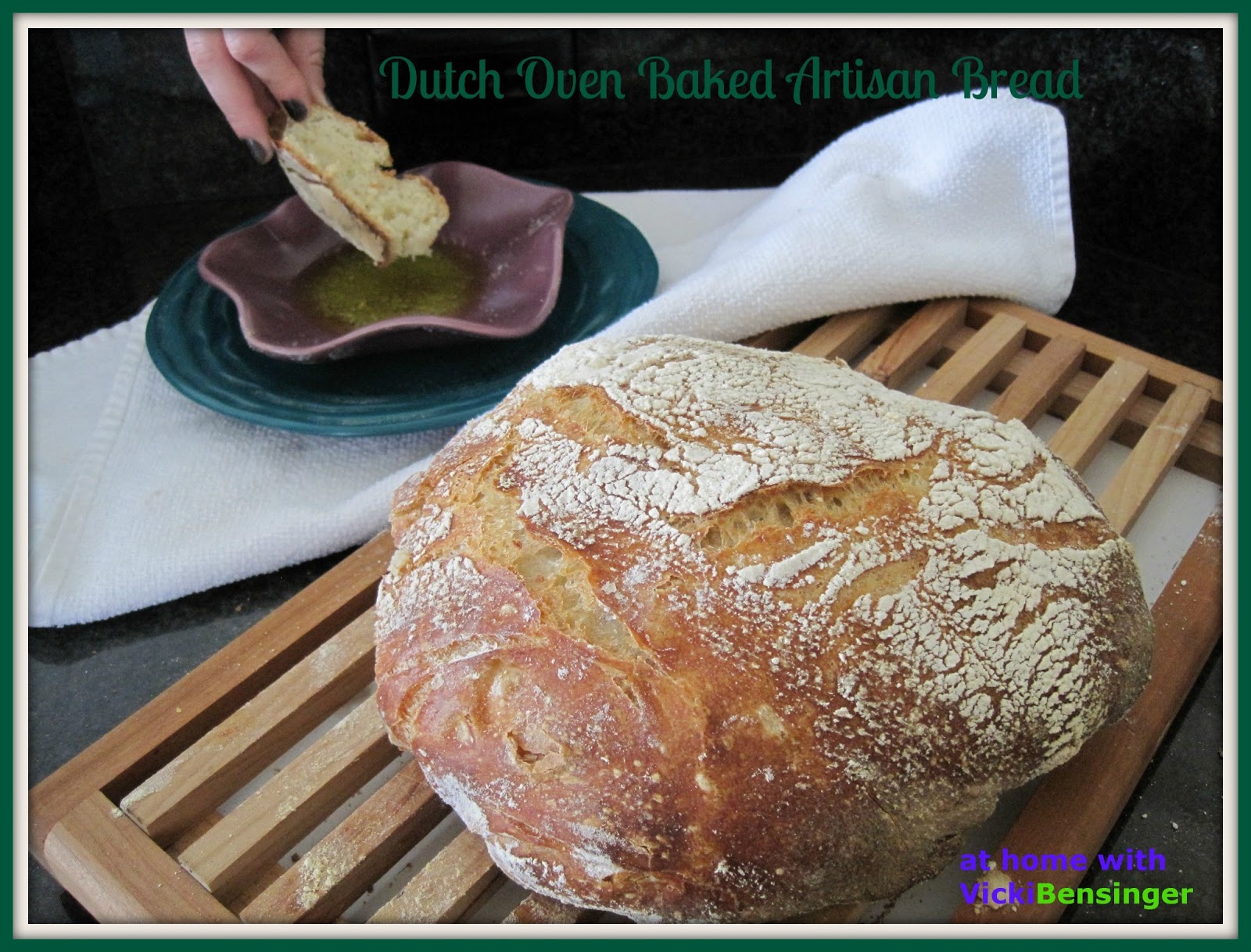This image features a close-up photograph of a freshly baked, circular homemade bread, with a light dusting of flour on its golden-brown crust. The bread rests on a wooden ventilated baking tray, adding a rustic touch to the scene. Overlaid in dark green text at the top, the image is labeled "Dutch oven baked artisan bread." On the bottom right, there is a purple text watermark that reads "@home with Vicky." To the left, a white kitchen towel drapes over the wooden rack. A hand is seen dipping a slice of this bread into a star-shaped, lavender-colored dish that likely contains olive oil or butter. This dish sits atop a green plate which is placed over the white kitchen towel in the top left of the image. The background is largely dark, creating a striking contrast that emphasizes the elements in the foreground.